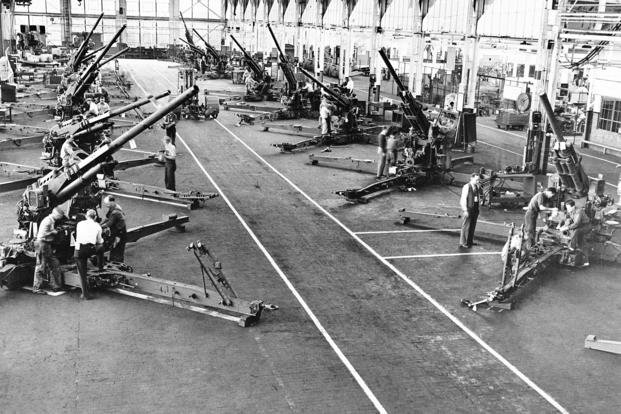This black and white photograph depicts a large indoor manufacturing facility, possibly serving a military purpose, as evidenced by the presence of massive artillery guns arranged in uniform rows. On the right side of the image, at least eight of these guns are neatly lined up, each with a base consisting of two long bars forming an X shape, supporting turrets with barrels angled upwards at approximately 65 to 70 degrees. Similarly, the left side showcases at least six additional guns, around which groups of men are huddled, either working on or observing the machinery. The facility features a central pathway marked with white lines, through which a vehicle is visible maneuvering. The high-ceilinged space, potentially enclosed with walls and glass sections, allows ample light to illuminate the scene, further highlighting the scale and meticulous arrangement of the equipment.